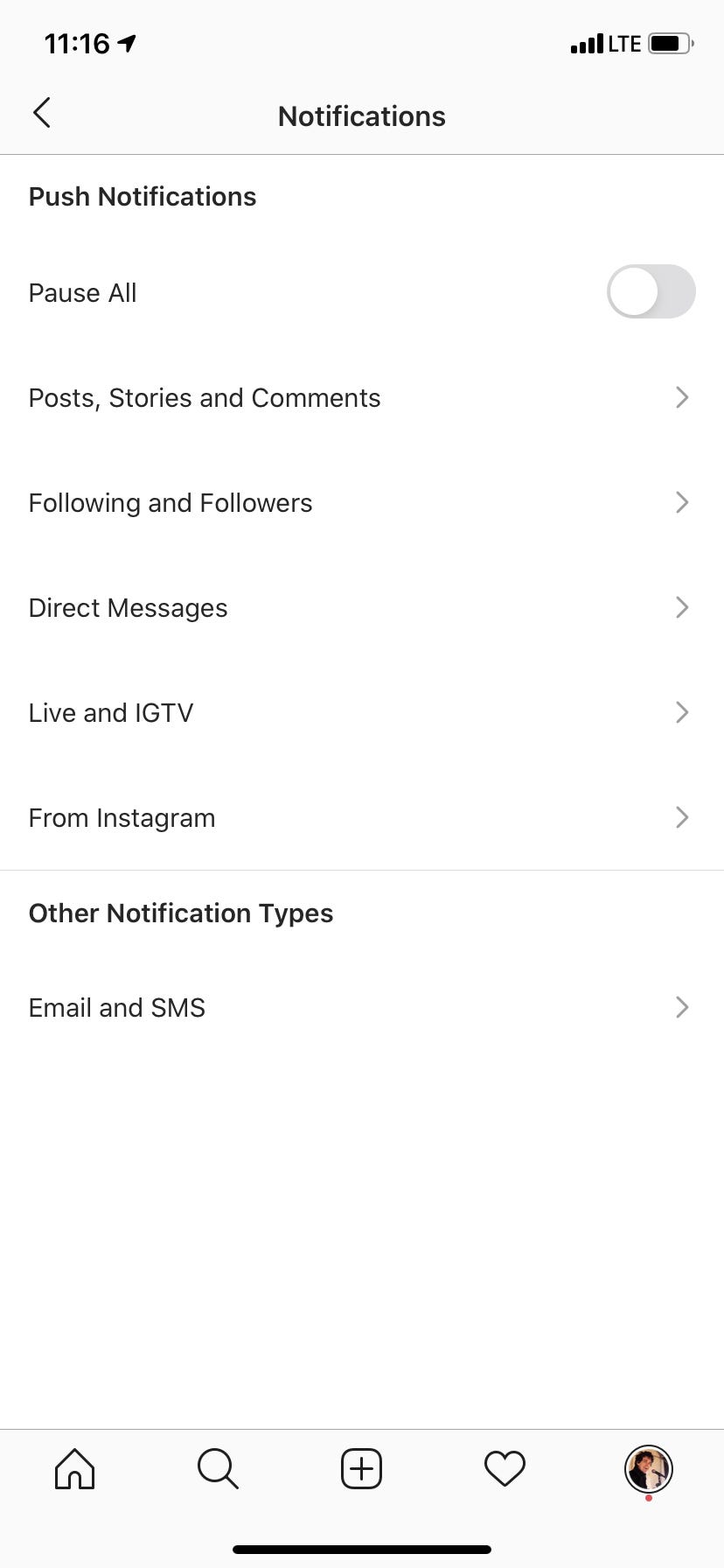The image depicts a mobile screen interface with a light gray notification bar at the top. The notification bar displays the time "11:16," along with icons indicating four bars of signal strength, LTE connectivity, and a battery level at approximately 75%. Below the notification bar, the screen has a white background starting with the header "Push Notifications."

Under the "Push Notifications" heading, there's an option labeled "Pause All" accompanied by a gray toggle switch positioned to the left. Following this, there are several notification categories, each with a greater-than symbol (indicating further options) to the right. These categories include "Post, Stories and Comments," "Following and Followers," "Direct Messages," "Live and IGTV," and "From Instagram."

Further down, another bold header reads "Other Notification Types," beneath which lies the option "Email and SMS." The screen has a considerable amount of white space below this section.

At the very bottom of the interface, a navigation bar includes icons for Home, Search (magnifying glass), Add (plus inside a square), Activity (heart), and Profile (profile picture).